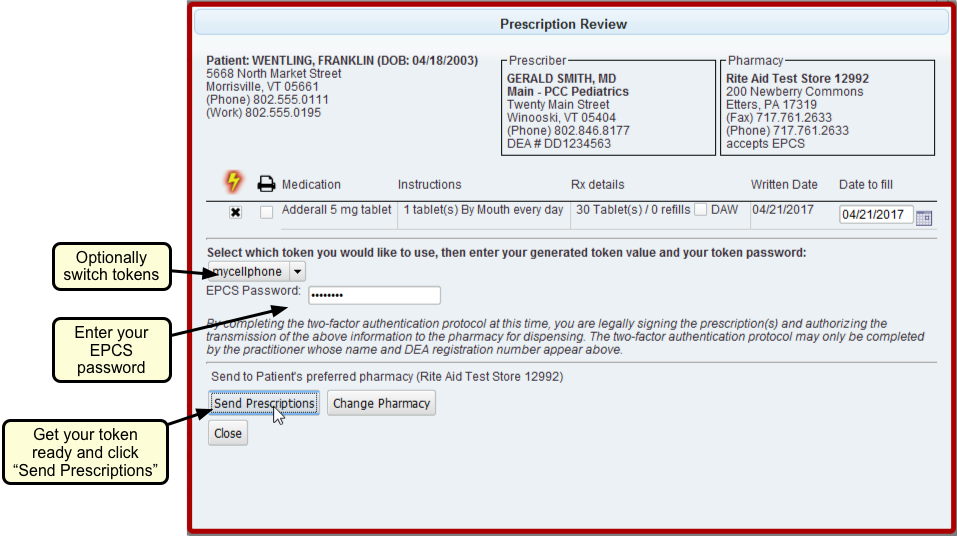This image is a detailed screenshot from a website with a very light sky blue background and a thin, brick-red border encircling a slightly wider-than-tall square. At the top center of the image, the header in gray font reads "Prescription Review." 

### Left Section:
On the left, the patient's details are listed:
- **Name:** Franklin Wentling
- **Date of Birth:** April 18, 2003
- **Address:** [Address is visible but not detailed here for privacy]

### Center Section:
In the center, prescriber information is provided:
- **Prescriber:** Gerald Smith, MD
- **Institution:** Maine PCC Pediatrics
- **Address:** [Prescriber’s address not detailed]

### Right Section:
On the far right, the pharmacy details are mentioned under the header "Pharmacy":
- **Pharmacy:** Rite Aid Test Store 12992
- **Address:** [Pharmacy address not detailed]

### Main Content:
Below these sections, the medication details are arranged from left to right:
- **Medication:** Adderall, 5-milligram tablets
- **Instructions:** [Instructions on how often to take it not provided]
- **Rx Details:** Includes the date the prescription was written, April 21, 2017.

Beneath the primary details, additional information is present but not specified in this description.

### Annotations:
To the left of the webpage, hand-drawn annotations and arrows direct attention to specific elements on the site. These notes include:
- "Optionally switch tokens"
- "Enter your EPCS password"
- "Get your token ready and click 'send prescriptions'"

This comprehensive layout ensures all critical information is easily accessible and visually organized.